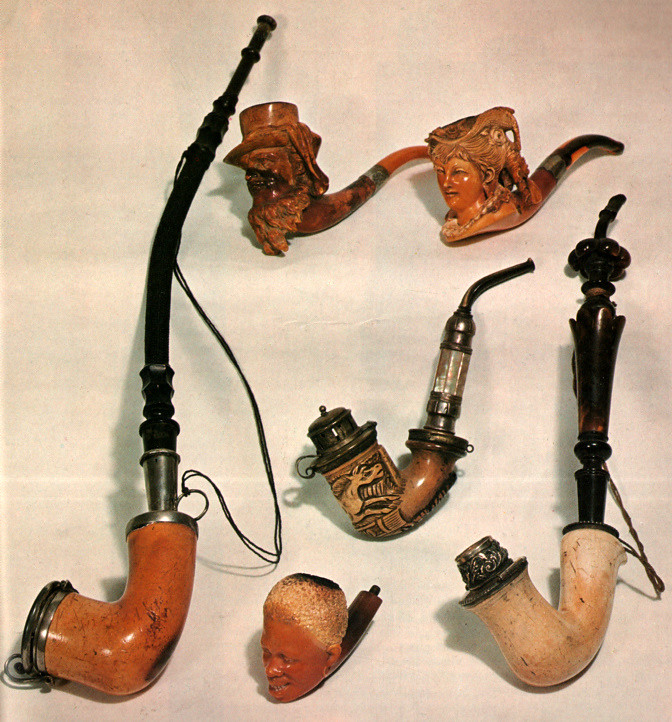The image showcases six distinct and unusual smoking pipes arranged on a tan background. Starting from the left, the first pipe is a British tan wood design with a black mouthpiece connected by a gray steel band, and features a round steel piece at the bowl's end. Moving upward, two pipes are designed to resemble human heads: the first is a British tan wood pipe intricately carved with the visage of a man wearing a top hat and sporting a beard, and the second is a female head carved from cognac wood, detailed with squinting eyes and pulled-back hair, with a black wooden mouthpiece. The central pipe is more elaborate, featuring an engraved horse and a removable cap at the bowl’s end, with a black mouthpiece connected via metal and steel fittings. The next pipe depicts the head of a Black man with an afro, made from cognac wood, and also ends in a black and tan mouthpiece. Finally, the last pipe on the right is a very light beige wood with a black mouthpiece. This collection includes pipes of varying lengths and intricate carvings, each with distinctive color patterns and design details, set against a light gray backdrop.